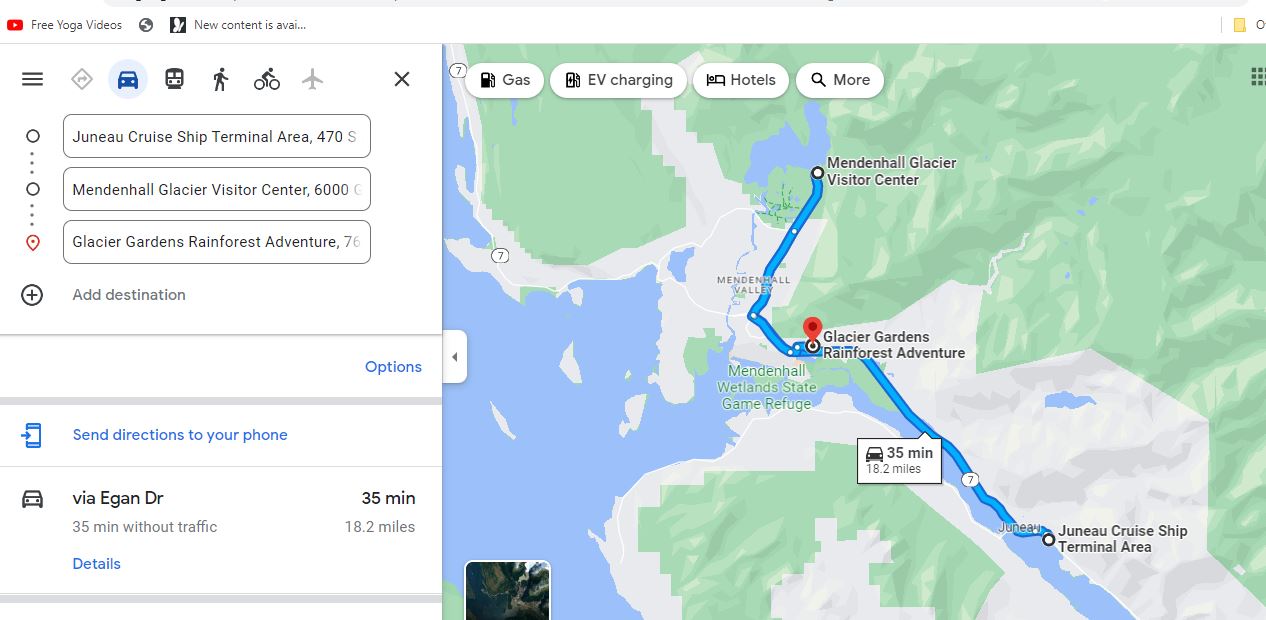The image is a detailed screen capture of a route planning interface, likely from Google Maps. The map illustrates a journey starting from the Juneau Cruise Ship Terminal in Juneau, Alaska. The planned route, highlighted in blue, projects a 35-minute drive covering 18.2 miles. Key stops along this picturesque route include the Mendenhall Glacier Visitor Center and the Glacier Gardens Rainforest Adventure. On the right side, the map features green topography for land and white areas indicating glaciers, with blue marking water bodies and the route. The driving option is highlighted among travel modes like public transport, walking, and biking. On the left, the itinerary is laid out, with specific directions via Eagan Drive, options to send the route to a phone, and an address snippet for Mendenhall Glacier Visitor Center. Above, icons indicating various functionalities and notifications, including 'Free Yoga Videos' and 'New Content Available,' are visible, along with a red arrow pinpointing the current location on the map.